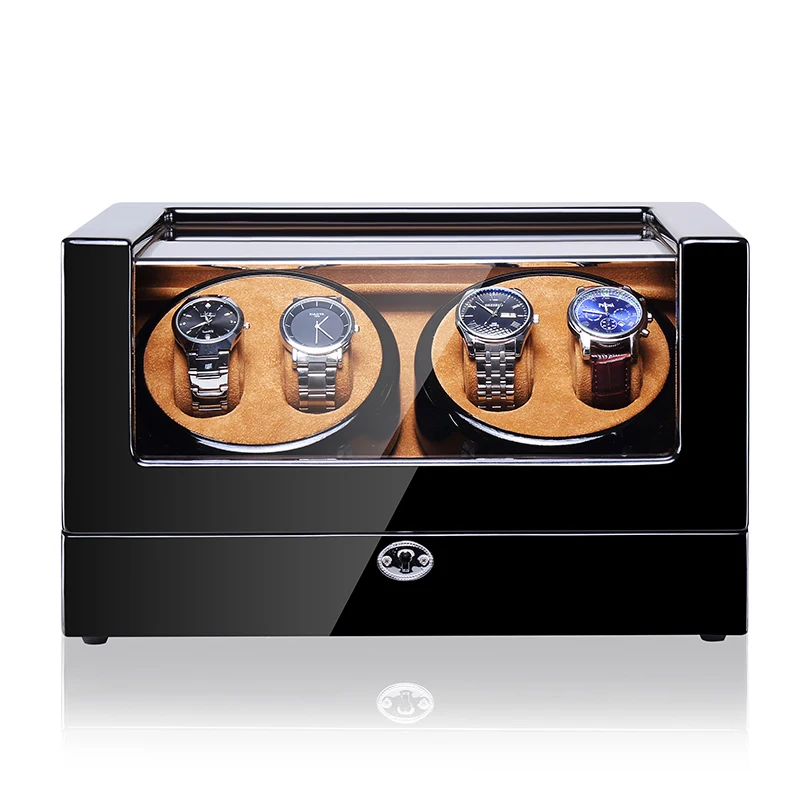This exquisitely stylized photograph showcases four wristwatches, meticulously arranged in a sleek black metallic display case with a transparent front panel. The glossy black box, featuring a silver keyhole at its bottom center, exudes a modern and sophisticated aura. Nestled inside the box are two tan-colored suede circular holders, each cradling two watches. On the left holder, the first watch boasts a black face with numerous secondary markers, while the adjacent watch shares a black face but with a simpler design. On the right holder, the left watch, also with a black face, presents intricate notch details, contrasting with the watch beside it, which displays a striking blue face and a leather-like strap. All the watches have silver bezels and are analog in function. The case itself sits on a lustrous white surface, creating a mirror-like reflection below, enhancing the overall elegance of the display. The photograph's background is flawlessly white, emphasizing the artificial, perfectly lit ambiance of the scene.